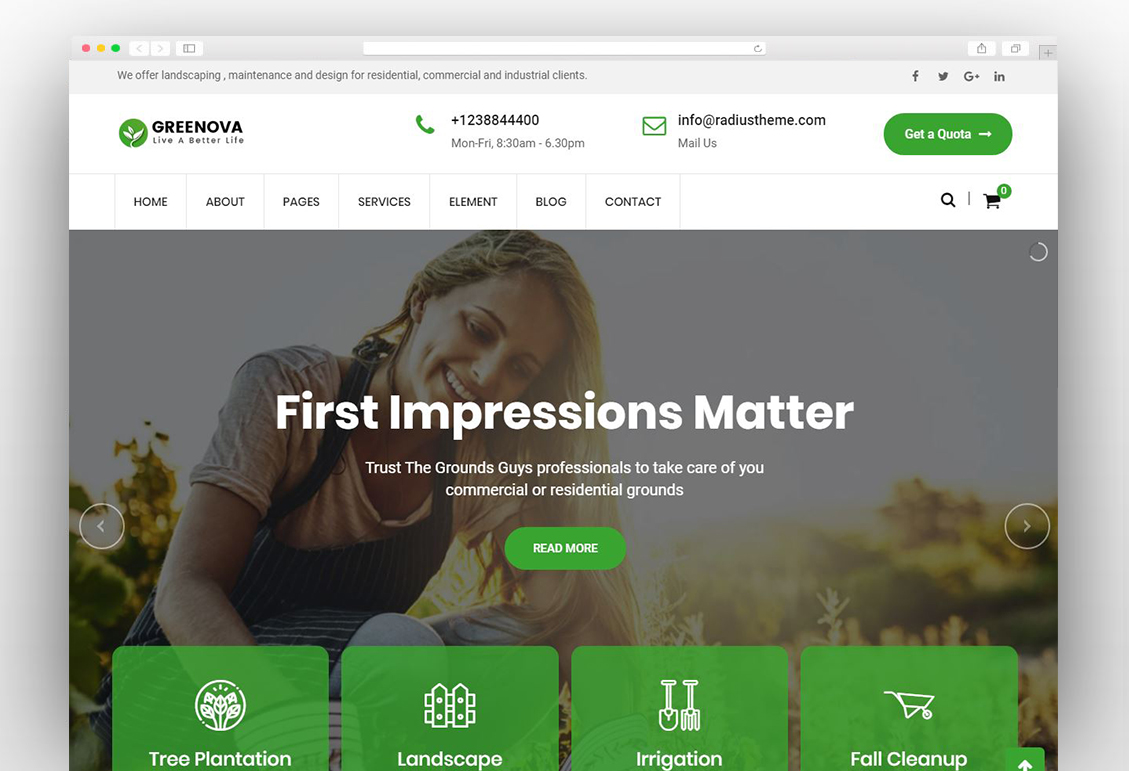A screenshot of the Green Nova website features a clean and organized design. In the top section, "Green Nova" is boldly written in black with the tagline "Live a Better Life" underneath. A small plant icon within a solid circle adds a touch of eco-friendliness to the presentation. The site navigation includes links to Home, About, Pages, Services, Element, Blog, Contact Us, and a Shopping Cart.

The main background image captures the essence of Green Nova’s mission, showcasing a person diligently planting. Overlaid text emphasizes the importance of first impressions with the statement, "First impressions matter. Trust the grounds guide professionals." The site promotes its services for both commercial and residential grounds maintenance, highlighting four key areas: Tree Planting, Landscaping, Irrigation, and Fall Cleanup. 

A "Read More" clickable link invites users to explore further. Below, additional information outlines the comprehensive range of services offered by Green Nova, including Landscaping, Maintenance, and Design for Residential, Commercial, and Industrial clients. Contact details, including a phone number and email information, provide easy ways for potential clients to reach out and start improving their grounds with Green Nova’s expertise.